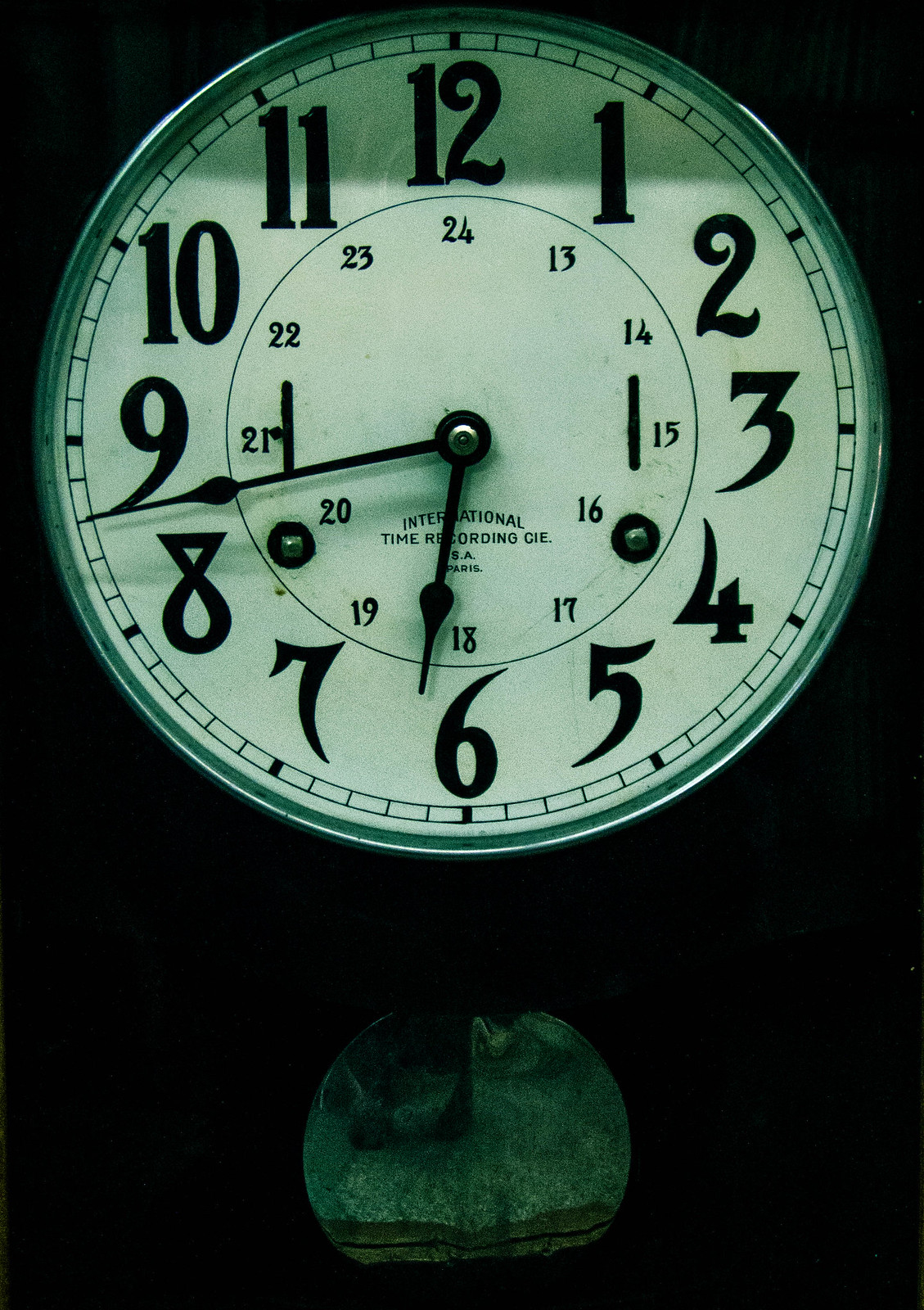The image depicts a round clock set against a very dark, almost black background, suggesting a dim or poorly lit environment. The clock features a thin silver metal border encircling a white face. It displays both regular and military time, with black numbers ranging from 1 to 12 for standard time and 13 to 24 for military time arranged in an inner circle. The elegant, slightly ornate font used for the numbers gives the clock a vintage appearance. The face of the clock is inscribed with "International Time Recording" followed by "CIE" or "GIE," and "S.A. Paris" beneath it. The clock also has two black hands indicating the time, which is approximately 6:43. Beneath the clock, there is a stone or rock that appears grayish-brown and black, although the exact details of its texture and shape are obscured by the darkness. There is some ambiguity about its color as it appears greenish to some viewers, indicating the lighting may be affecting the perception of its hues.